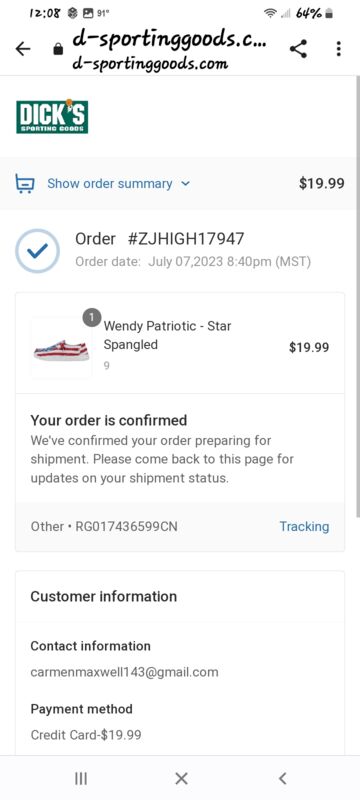Here is a clean and detailed caption for the image described:

---

This image is a screenshot from a mobile device, showcasing a completed order page from Dick’s Sporting Goods' website. The background of the page is white, and the web address is visible at the top alongside a black back arrow, a share button, and another button in the top right corner. 

Just below, there is a teal green banner with "Dick's Sporting Goods" written in white text. Below this banner, a drop-down box labeled "Show order summary" is displayed with the price of $19.99 USD to its right. 

Further down, the details of the order are shown: a check mark indicates the order has been placed, along with an order number and the time of order placement - July 7th, 2023, at 8:40 p.m. Mountain Standard Time. The product ordered is described as "Windy Patriotic Star-Spangled Shoes" in size 9. 

Beneath these details, the order confirmation status is displayed as "Confirmed." The customer’s contact information field is blank, but their email is shown. The selected payment method is a credit card.